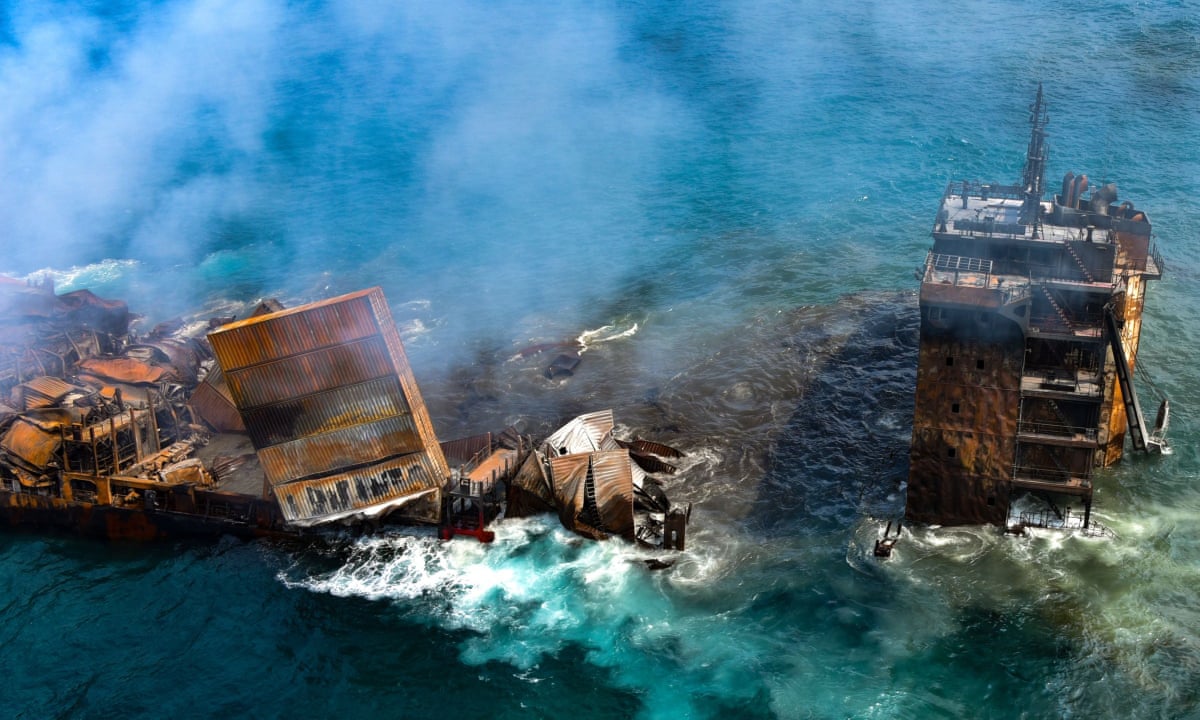This is a detailed aerial photograph depicting the aftermath of a devastating explosion on an offshore oil drilling rig. The rig is partially submerged in a shallow section of the ocean, with sections of it still visible above the water. The massive structure on the right, likely the bridge and manning tower, stands tall with numerous steps leading upwards, despite the extensive damage. The paint on this section is burnt orange and peeling away, hinting at the intensity of the blaze that once engulfed it. 

To the left, the rest of the drilling platform lies in chaotic disarray, with large machinery and metal pieces haphazardly strewn about. Some components appear crumpled and heavily burnt, while others are rusty, contributing to the overall apocalyptic scene. Thick white smoke and steam rise from various parts of the wreckage, suggesting that the fire has only recently been extinguished or is still smoldering. A distinct brown liquid, likely oil, contaminates parts of the otherwise blue ocean, indicating a significant oil spill.